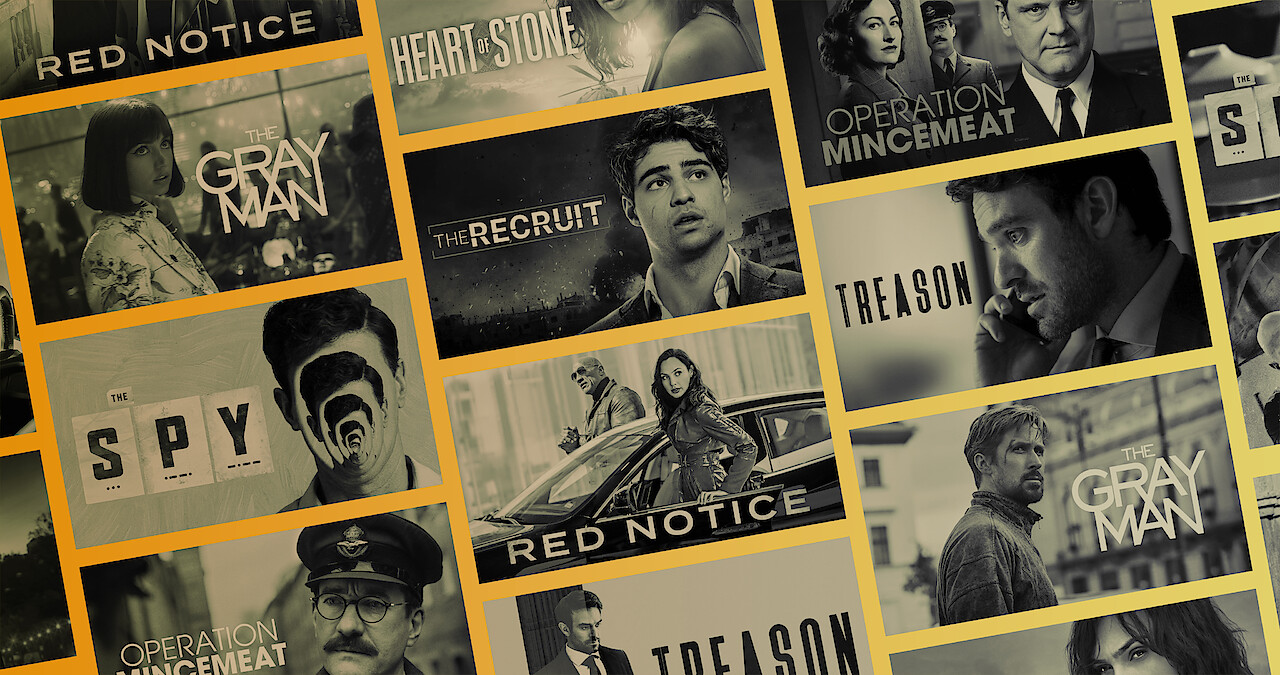The edited image exhibits a collection of black and white movie and TV show posters, each precisely organized into staggered columns, all angled slightly towards the top left. Distinguished by a vibrant border, which shifts from a warm dark orange on the left to a bright yellow on the right, creating a vivid contrast against the monochromatic posters. Featured prominently are titles like "The Spy," "The Gray Man," "Red Notice," "Operation Mincemeat," "Treason," "The Recruit," and "Heart of Stone," each repeated in different orders throughout the columns. "The Spy" is notable for depicting a man's face within faces, and "Operation Mincemeat" showcases a police officer with glasses. "Heart of Stone" appears truncated at the top of the second column, while "The Recruit" and "Red Notice" show a young man and a duo near a car, respectively. The various posters, bordered in gold, aim to highlight the platform's or channel’s featured content in a visually striking manner.